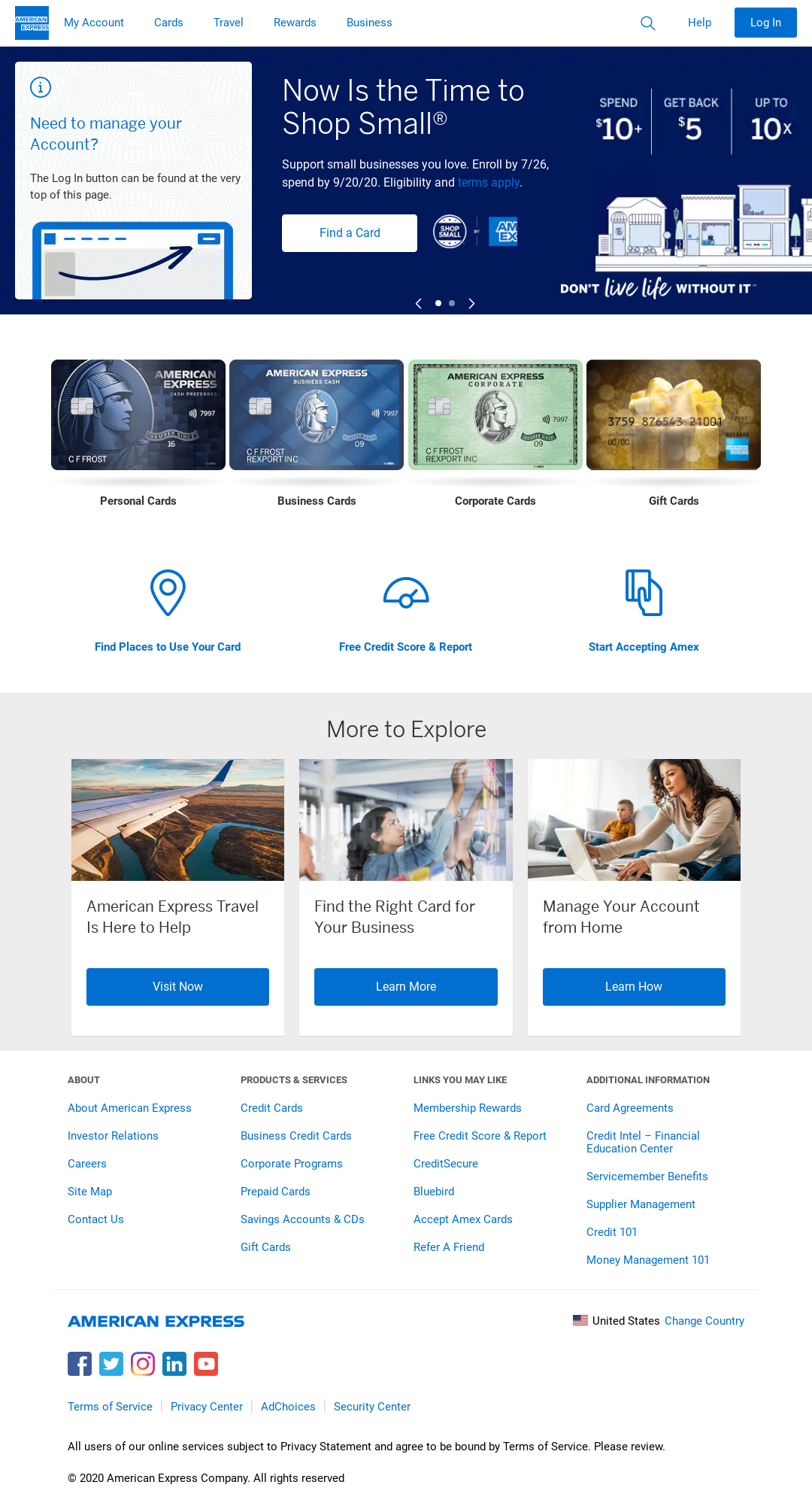Screenshot of the American Express Website

The screenshot captures the American Express website, showcasing various sections and options for users. At the top left, a blue bar prominently displays "American Express" in blue letters with a white outline. To the right of this logo, the menu includes options: "My Account," "Cards," "Travel," "Rewards," and "Business," along with icons for search (magnifying glass), "Help," and "Login."

On the left side, a white square reads "Need to Manage Your Account? The Login button can be found at the very top of this page." An illustration of a computer monitor with a black arrow points towards the Login button located at the top right.

A prominent message encourages users to "Shop Small" and support small businesses. It notes an enrollment period ending on 7/26 and a spending deadline of 9/2020. Terms and eligibility apply. Customers are invited to spend $10 or more and get $5 back, up to ten times.

The next section features a drawing of quaint small businesses alongside the phrase "Don't Live Life Without It." Below this, images of different American Express cards are displayed:
- A gray and black card labeled "Personal Cards."
- A blue card labeled "Business Cards."
- A green card labeled "Corporate Cards."
- A gold card adorned with a gift box and bow, labeled "Gift Cards."

Further down, options include "Find Places to Use Your Card," "Free Credit Score and Report," "Start Accepting Amex," and various exploratory links like "American Express Travel is here to help," "Find the right card for your business," and "Manage your account from home."

The bottom section houses multiple links categorized under headings such as:
- About: Including "About American Express," "Investor Relations," "Careers," and "Contact Us."
- Products and Services: Listing "Credit Cards," "Business Credit Cards," "Corporate Programs," "Prepaid Cards," "Savings Accounts and CDs," and "Gift Cards."
- Links You May Like: Featuring "Membership Rewards," "Free Credit Score and Report," "Credit Secure," "Bluebird," "Accept Amex Cards," and "Refer a Friend."
- Additional Information: Including "Card Agreements," "Credit Intel Financial Education Center," "Service Member Benefits," "Supplier Management," "Credit 101," and "Money Management 101."

Lastly, the footer contains icons for American Express’s social media on Facebook, Twitter, Instagram, LinkedIn, and YouTube. It also includes links for "Terms of Service," "Privacy Center," "Ad Choices," and "Security Center." A note informs users that they are subject to the privacy statement and Terms of Service upon using the site's services. The copyright note at the bottom states, "2020 American Express Company. All Rights Reserved."